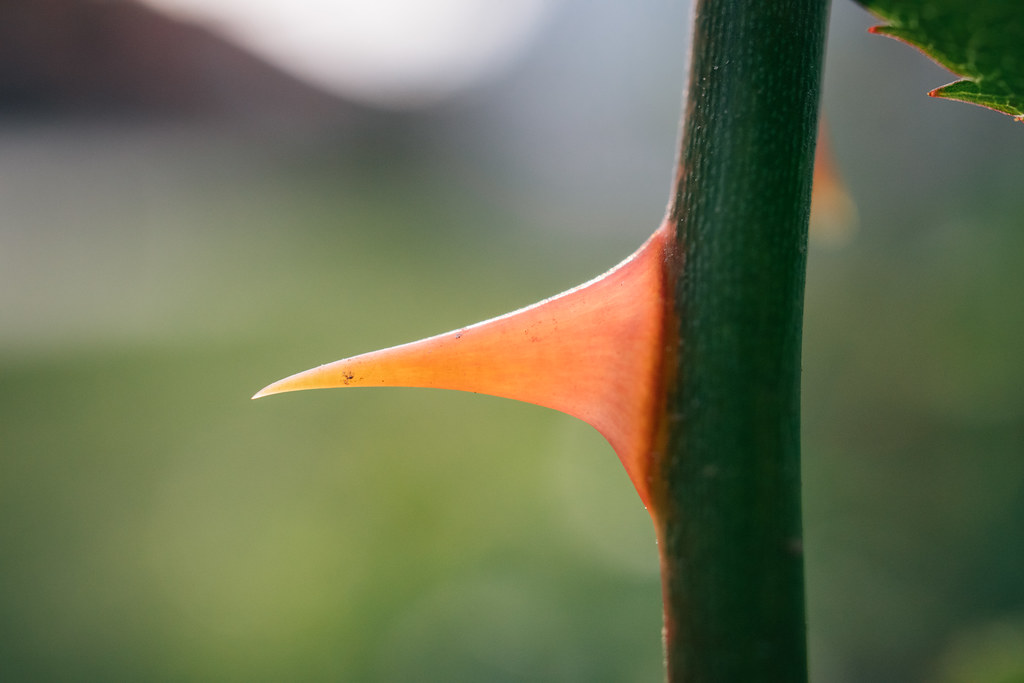This photograph features a close-up of a thorn protruding from a green vine, emphasized by a sharply blurred background of varying shades of green and gray. Centralized slightly to the right, the vine extends vertically, presenting a detailed triangular thorn jutting out to the left. The thorn exhibits a gradient of colors, transitioning from pinkish and grayish tones near its base to a dark orange near the tip, which curves subtly downwards. In the upper right corner of the image, a small leaf with red-tipped edges provides a hint of natural detail. The blurred backdrop effectively draws focus to the intricate textures and colors of the thorn and vine, creating a striking visual contrast.